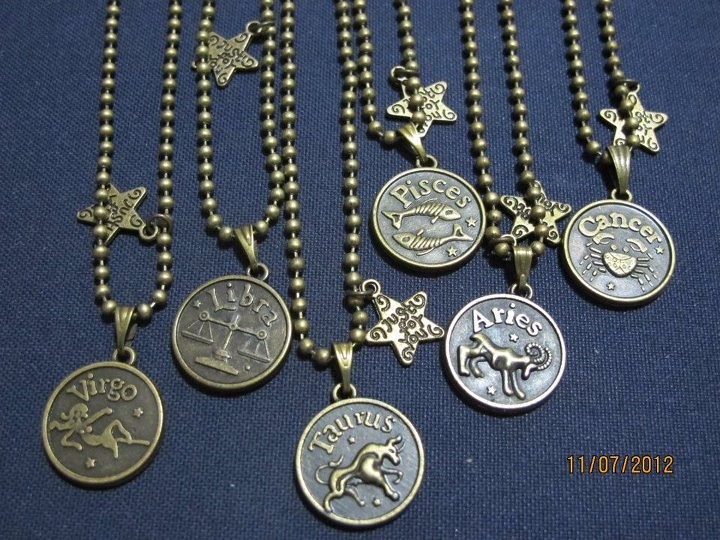This landscape-oriented photograph features a close-up view of several necklaces, each adorned with circular medallions that depict different astrological signs. The medallions, crafted from a brass-like material, hang from silver ball chains that are uniformly arranged. Each medallion resembles a coin with raised designs and inscriptions denoting the various astrological signs. Against a dark blue, denim-like background, the necklaces cascade downwards. Notably, at the bottom right corner of the image, the date "11/07/2012" is superimposed in orange.

From left to right, the displayed medallions represent Virgo, Libra, Taurus, Pisces, Aries, and Cancer. The Virgo medallion bears the image of a reclining woman, Libra features balancing scales, Taurus displays a bull, Pisces has two fish, Aries shows a ram, and Cancer is adorned with a crab. Additionally, small, flat star-shaped metal charms dangle from each chain with the inscription "Just for you."

The arrangement of the medallions varies in height across the image, creating a staggered, multi-row layout. Virgo, on the far left, is slightly higher than the neighboring Libra and Aries medallions, while Taurus is positioned lowest in the bottom center. Pisces and Cancer occupy the highest positions in the top row, creating an eclectic yet balanced visual.

This detailed snapshot captures the intricate craftsmanship of the medallions and the thoughtful arrangement of the necklaces, all set against a textured backdrop, emphasizing both the aesthetic and the thematic elements of the astrological signs.